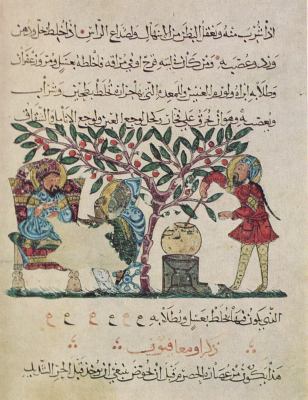This image appears to be a very old painting with an aged cream background. At the top, there are four lines of text written in black, which is likely in a language similar to Arabic. The central part of the image portrays a scene with several elements: on the left, a man is depicted sitting on what looks like a red throne. In the middle, an olive tree is prominently displayed, branching out with green leaves and red berries. To the right of the tree, there is a black crate or box holding a fishbowl-shaped container. Another man, wearing a red top and yellow tights, stands next to it, stirring the contents of the container with a stick; he has a long, dark braid running down his back. At the bottom, the image is finished with three additional rows of text.